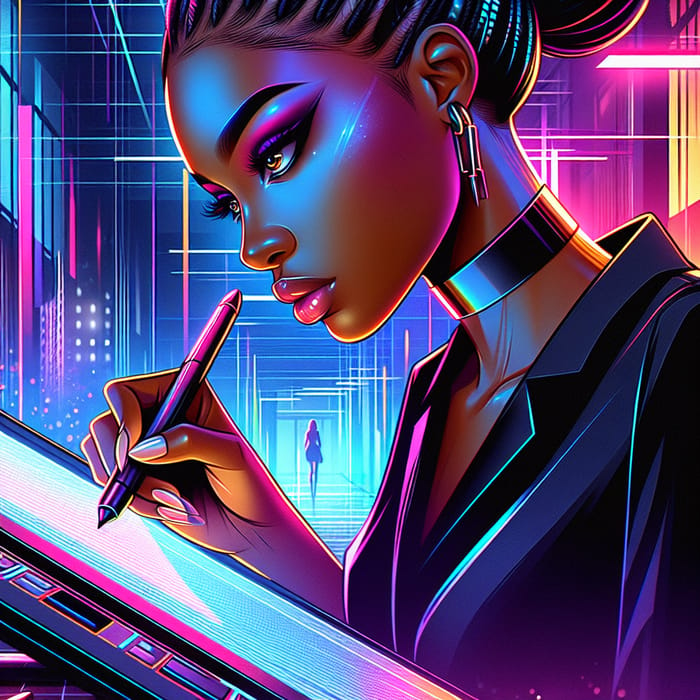In this stunning, futuristic artwork, an AI-generated or graphic-designed image depicts a beautiful Black woman with her hair styled in intricate braids pulled into a bun, complete with meticulous baby hairs. She stands in front of a vividly glowing neon background dominated by synthwave hues of pink and cyber blue, contributing to a surreal, otherworldly atmosphere. The left side of the backdrop reveals a tall building, adding to the urban, high-tech setting.

The woman is intently focused on a futuristic tablet in her right hand, her gaze unwavering as she appears to draw with a stylus. Despite the tablet seemingly displaying just a wallpaper, the positioning suggests she is deep in creative work. She wears a dark purple blazer, complemented by pink lipstick, and purple-pink eyeshadow that harmonizes with the overall color scheme.

Her accessories further emphasize the futuristic theme: she has long square metallic earrings and a matching collar necklace that enhance her sophisticated attire. Additionally, she dons a choker around her neck. Her facial features are striking, characterized by long eyelashes, well-defined eyebrows, and a sharply defined jawline. The image's depth is enhanced by another woman walking away in the background, contributing to the sense of a dynamic, bustling environment. The entire scene radiates an album cover aesthetic with its vivid colors and cyberpunk vibe, making it visually mesmerizing and intricately detailed.